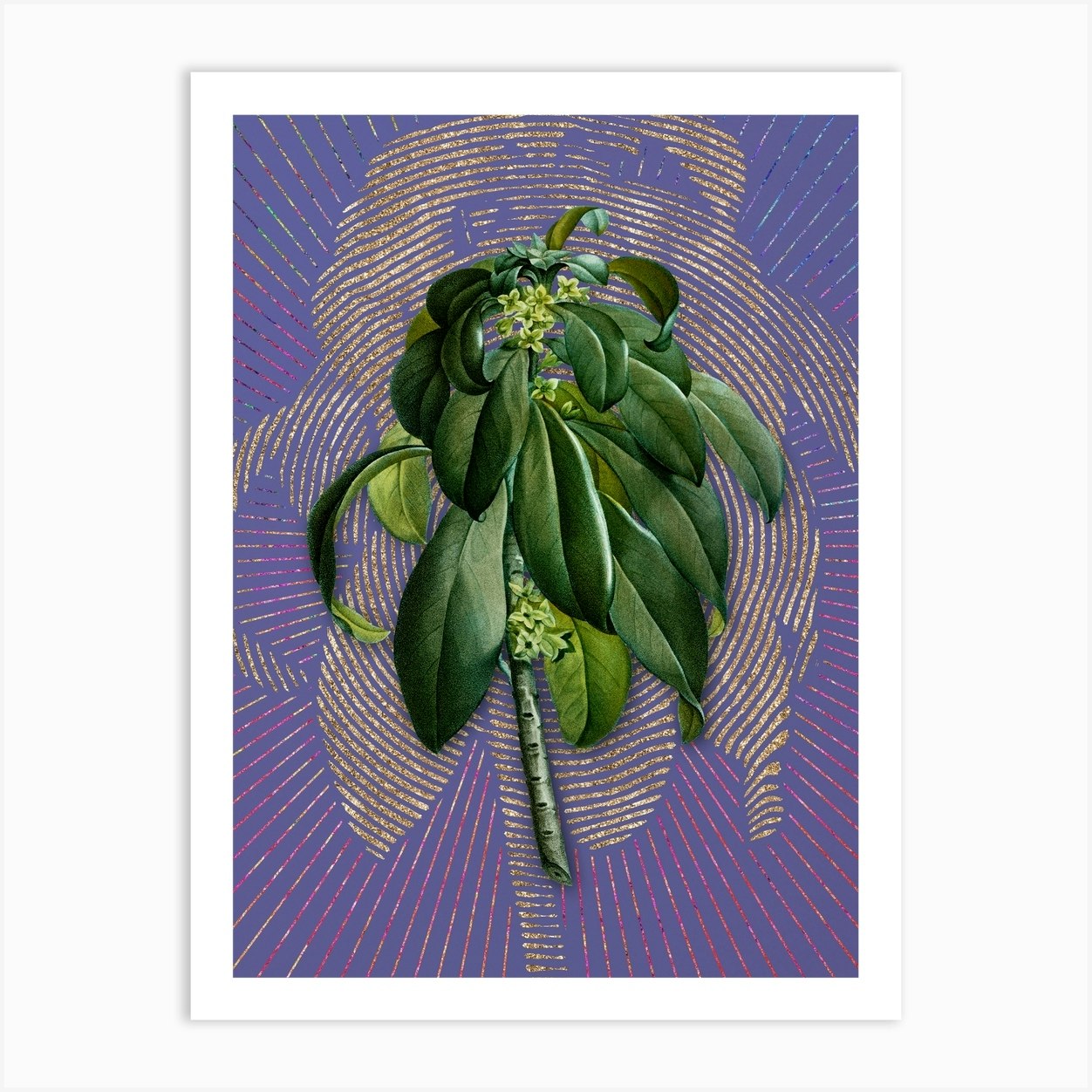This detailed digital illustration depicts a glossy, dark green tropical branch at its center. The branch is adorned with large, shiny leaves reminiscent of magnolia leaves, folding down in long, skinny shapes. Clusters of light greenish-yellow flower buds emerge towards the top and bottom of the branch. The background is a deep purple, featuring a larger, posterized version of the central image in a tannish gold hue. This artistic choice creates a mimicry effect, with golden lines tracing the branch and leaves, enhancing the contrast against the rich purple backdrop. The entire scene is framed in white, highlighting the intricate design and naturalistic elements within the decorative composition.